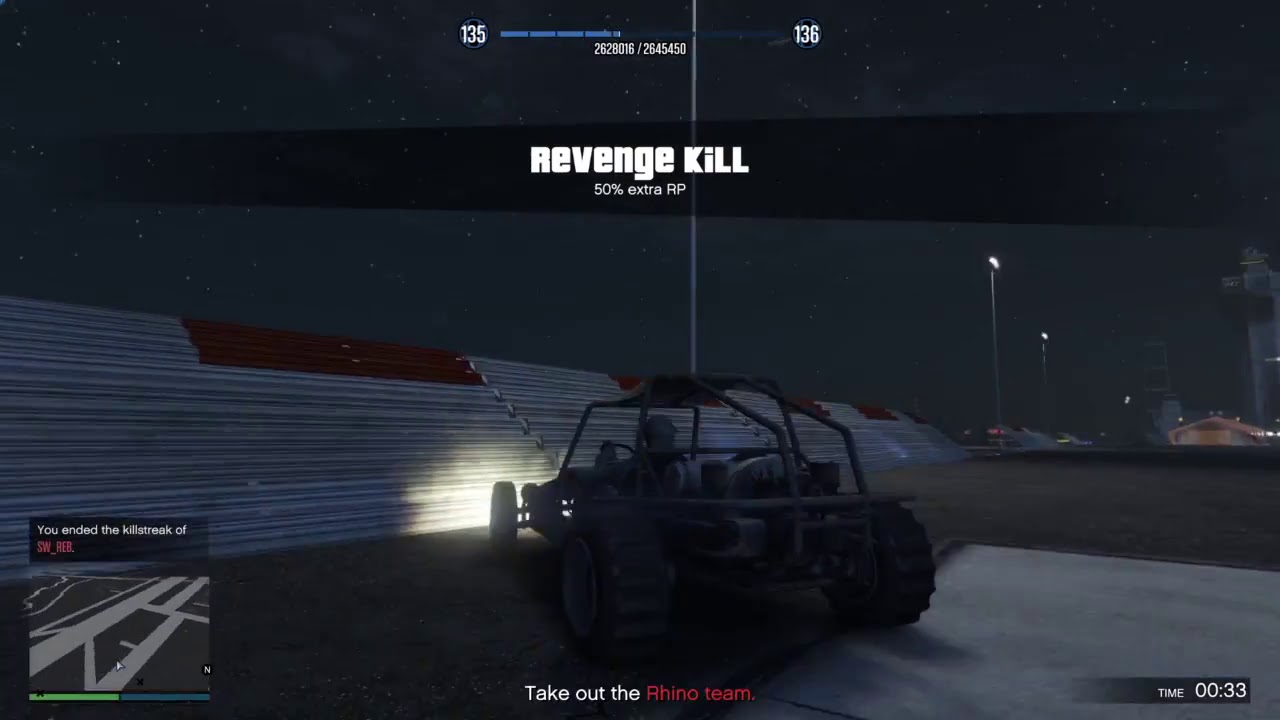The image is a dark, night-time screenshot from inside a video game, showcasing intense action on a dirt track stadium. The prominent vehicle, an off-road all-terrain vehicle equipped with a roll cage and thick tires, is driving away from the camera towards a diagonal wall and ramps. Illuminated by its own headlights, the vehicle highlights the surrounding terrain including grandstands, several streetlights, and possibly some homes and trees in the background, although these details are faint due to the darkness. The driver of the vehicle is visible, maneuvering towards the adversaries in the game. 

Key elements of the interface are overlaid on the image: At the top, there's a health bar and some numerical indicators. The bottom left features a mini-map showing the vehicle's position and trajectory, while the bottom right displays a timer set at 00:33. Central upper text reads "Revenge Kill," and below the vehicle, the objective "Take out the Rhino team" is prominently visible. These details contribute to the immersive, high-stakes environment typical of action-packed racing or combat gaming scenarios.